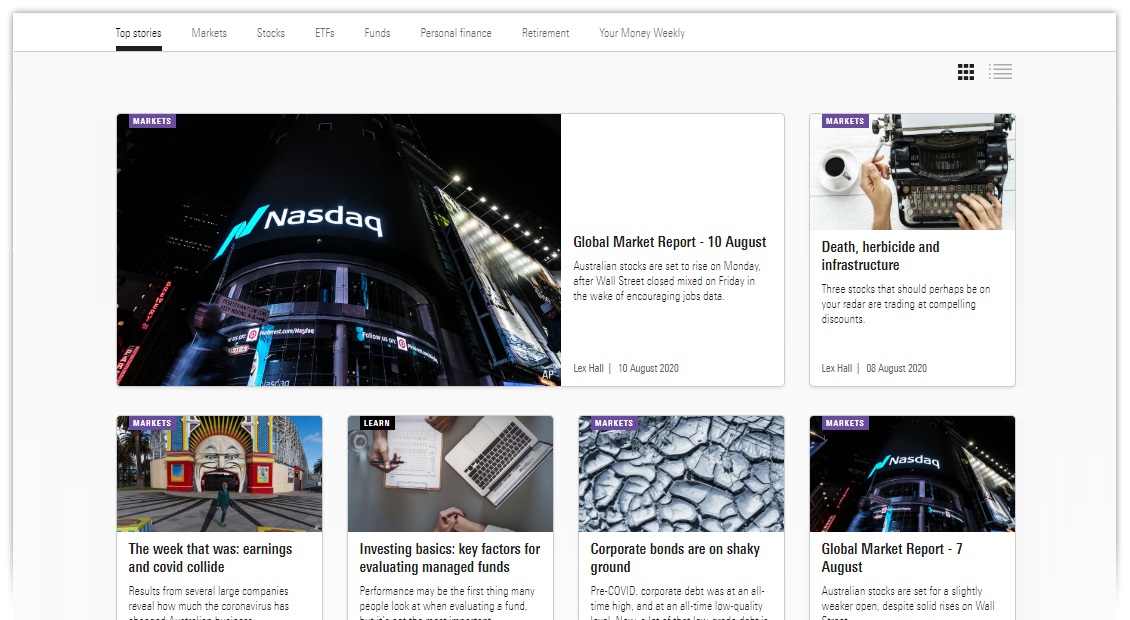This is a screenshot from a news website featuring a white navigation bar at the top with tabs for "Top Stories," "Market Stocks," "ETFs," "Funds," "Personal Finance," "Retirement," and "Your Money Weekly." The current selection is on "Top Stories." In the right-hand corner of the navigation bar, there's a grid icon to toggle between grid and list views, and the display is currently set to grid view.

The main article highlighted is a global market report dated August 10, 2020. It features a headline stating that Australian stocks are expected to rise on Monday after Wall Street closed mixed on Friday, following encouraging jobs data. The article, authored by Lex Hall, is accompanied by an image of the Nasdaq.

To the right of this main article, there is another feature titled "Death, Herbicide, and Infrastructure: Three Stocks to Watch." This article, also authored by Lex Hall on August 8, 2020, includes an image of a typewriter with a person's hands on it, suggesting a focus on detailed analysis.

Below these articles are additional pieces, including:
- "The Week That Was: Earnings and COVID Collide," featuring an image of a building.
- "Investing Basics: Key Factors for Evaluating Managed Funds," showing a picture of a laptop with someone taking notes.
- "Corporate Bonds on Shaky Ground," illustrated with an image of cracked ice.
- Another "Global Market Report" from August 7, featuring a similar image of the Nasdaq.